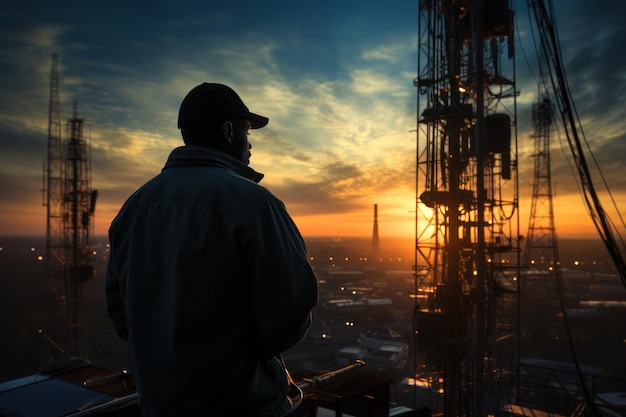In this evocative nighttime scene, a man wearing a blue jacket with the collar turned up and a black baseball cap stands silhouetted against a breathtaking sunset. The sky above transitions from deep blue at the top, scattered with separated clouds, to a brilliant orange and red nearer the horizon where the sun is setting. He is positioned amidst a network of industrial equipment—likely an oil rig—characterized by towering metal structures, intricate wiring, and machinery. His attention is fixed on the cranes and the complex array of cables before him. In the distance, faintly illuminated buildings and low hills frame the darkened landscape. The entire setting is suffused with a sense of quiet contemplation as the man, whose back is turned to the viewer, gazes out over the scene, merging his silhouette with the dimming light of dusk.